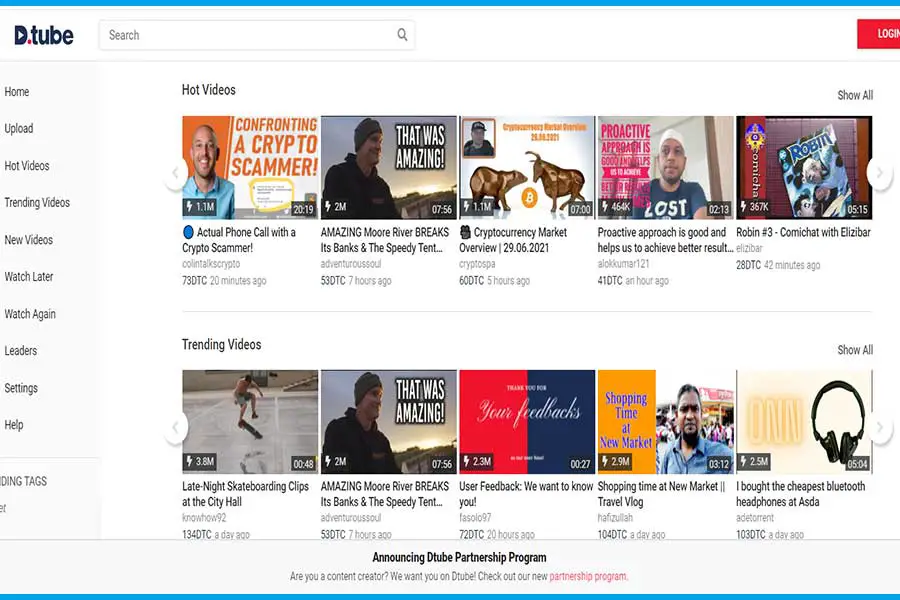The image showcases a YouTube-like webpage interface. At the very top, a narrow blue bar stretches horizontally from edge to edge. Below this, on the left, the logo reads "dotTube." 

To the right of the logo, there is a search bar prominently displayed. Further to the right, a "Log In" button in red stands out against the white background.

The main content area is divided into two distinct sections. The top section, labeled "Hot Videos," features a horizontal row of five video thumbnails. 
- The first thumbnail is titled "Actual Phone Call with a Crypto Scammer."
- Next to it is "Amazing More River Breaks and Banks."
- The third video is "Cryptocurrency Market Overview."
- Following this is "Proactive Approach and How it Helps Us Achieve Better Results."
- The last video in this row is "Comedy Chat with Elisabar," labeled as Robin #3.

Below this, the "Trending Videos" section displays another row of five video thumbnails.
- The first video on the left is "Late Night Skateboarding Clips at the City Hall."
- Next is "Amazing More River Breaks and Banks and Speedy Tent."
- The third video, titled "User Feedback, We Want to Know You."
- Adjacent to it is "Shopping Time and New Market Travel Vlog."
- The final video in this category is "I Bought the Cheapest Bluetooth Headphones at ASDA."

The overall background of the page is white, with additional categories listed on the left-hand side. Another blue bar runs horizontally along the bottom of the image, mirroring the one at the top.